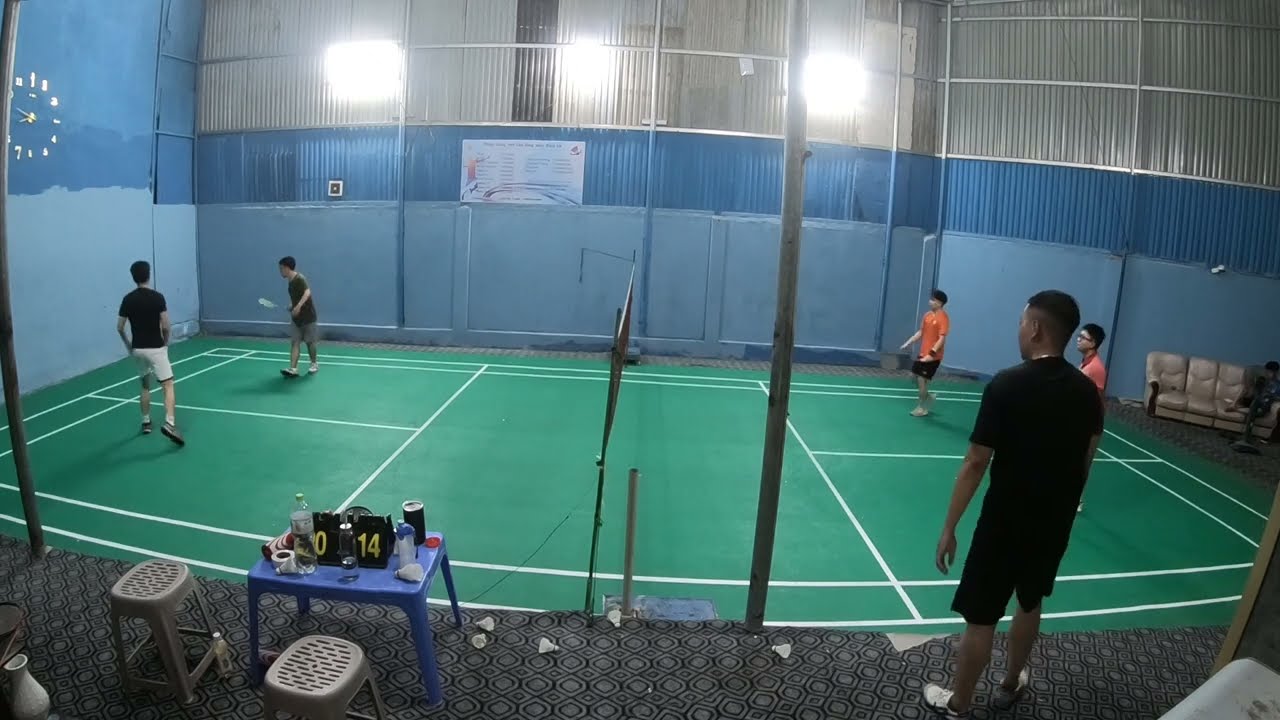This horizontally aligned rectangular image captures a game taking place on an indoor court, which appears to be pickleball or badminton. The court, located inside a building with gray walls adorned with layered fabric—blue at the bottom and beige above—is green with white lines, resembling a smaller tennis court. In the middle of the court, a net is implied, though not visible. 

On the left side of the court, two young male players dressed in black t-shirts and shorts, varying between white and gray, are gearing up to face their opponents. On the right side, two men clad in orange t-shirts and black shorts stand ready, facing their opponents. Both teams have players with short dark hair. 

In the foreground, a man in a black t-shirt and black shorts observes the game intently. He stands on a gray and black diamond-patterned carpet or rubber area. This foreground area also features two short gray plastic stools and a small blue plastic table, likely hosting miscellaneous items, including water bottles. Additionally, a clock is visible in the upper left corner of the wall, and windows at the top of the wall offer a space for observers. On the opposite side of the court, a white sofa provides further seating options.